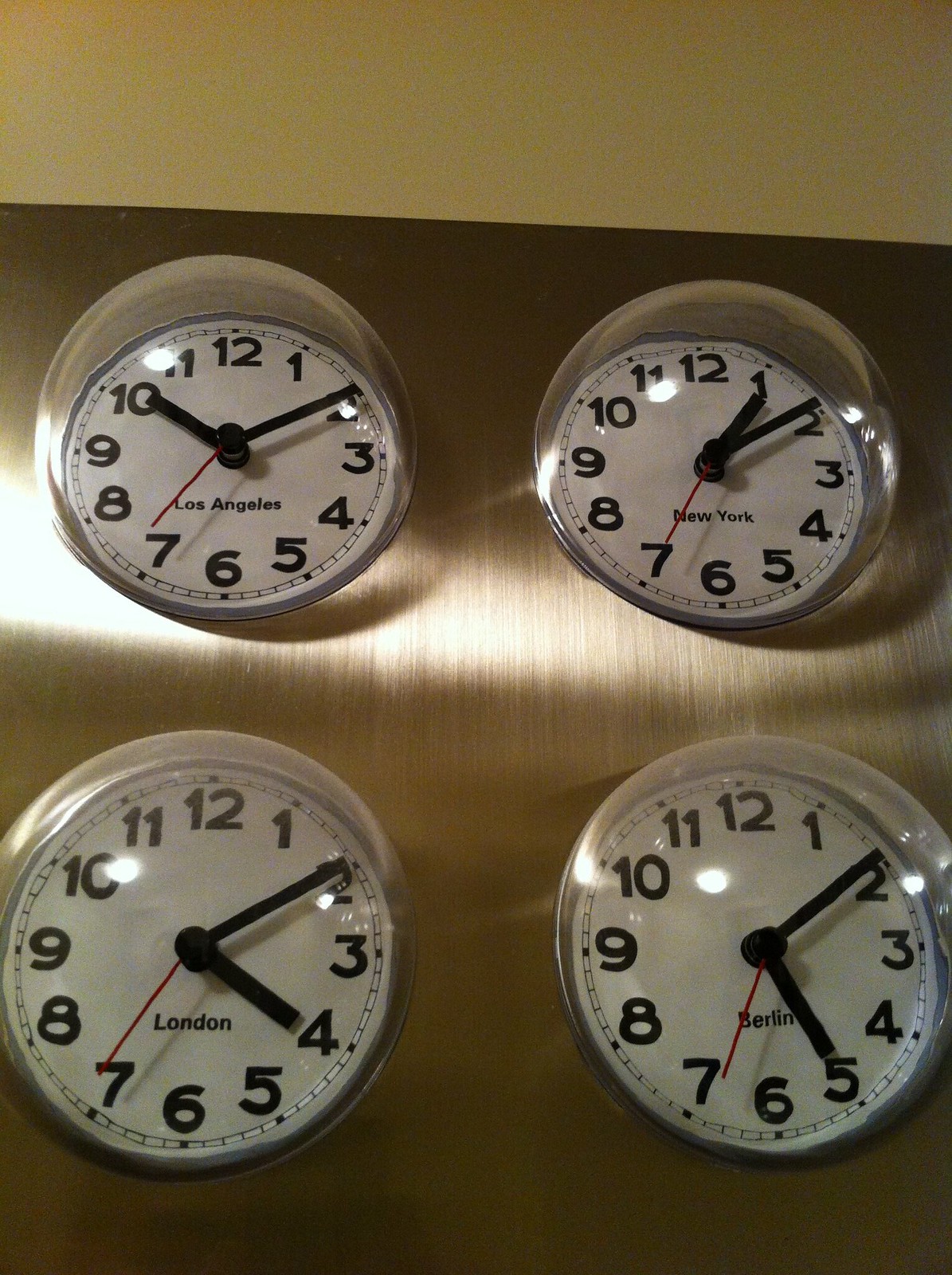This detailed color photograph displays four classic-style clocks arranged in a square formation against a stainless steel background, which extends three-quarters up the image and gives way to a yellowish light on a wall behind. Each clock features a white face with prominent black numbers and hands, a red second hand, and is encased in a clear glass dome. The upper left clock indicates the time in Los Angeles as 10:10, while the adjacent clock to the right shows the New York time as 1:10. Below these, the lower left clock reads 4:10 for London, and the lower right clock displays 5:10 for Berlin. All clocks are labeled accordingly with black text.